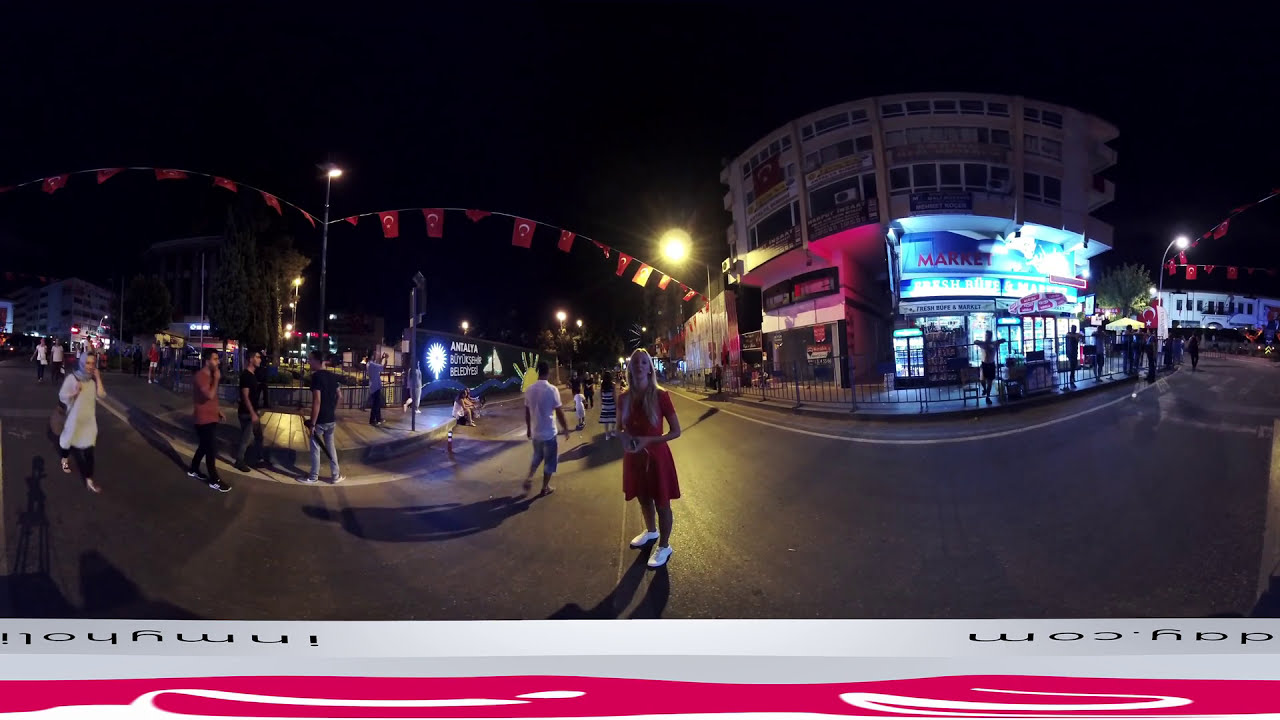In this vibrant night scene taken with a fisheye lens, a bustling city square is alive with nightlife. At the forefront stands a young woman with long blonde hair, dressed in a red summer dress and white sneakers, posing confidently for the camera. She holds a small bag or camera, and an illuminated street lamp behind her casts a bright light, highlighting her presence. The setting seems festive, with red and yellow flags draped across the street and neon signs adding splashes of color. A distinctive sign behind her reads "Antalataya" in a foreign language, contributing to the warm, possibly summer atmosphere, evidenced by people in a mix of shorts and jeans. Market stalls and shops line the right side of the street, and the URL "inmyholiday.com" appears faintly at the bottom of the screen, suggesting the image might be part of an online travel diary. The street is noticeably clear of cars, enhancing the scene's lively pedestrian energy, with people milling around, including groups of men and women, some of whom appear to be also enjoying the night out.